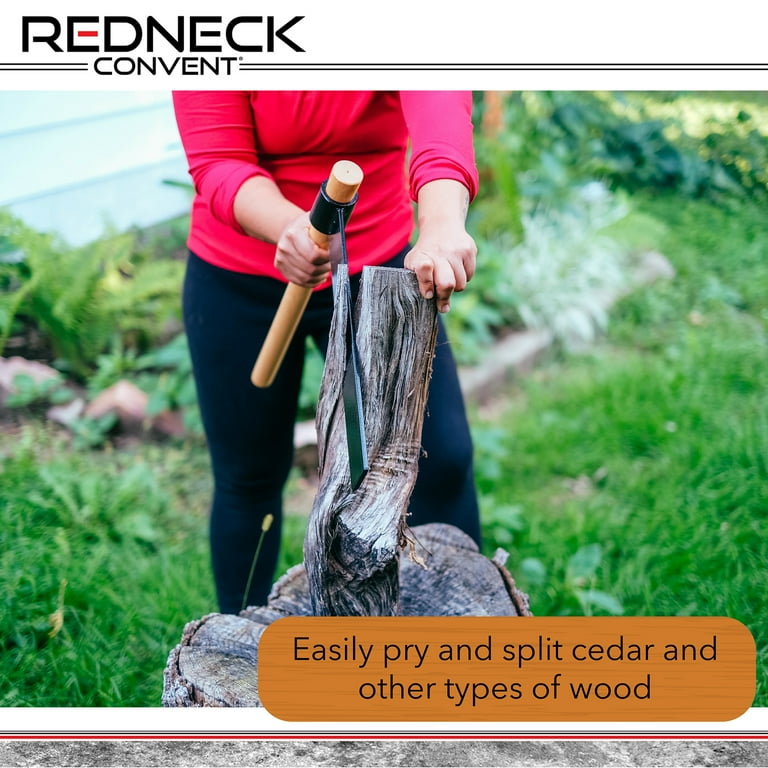This is a detailed photograph ideal for a sales advertisement, featuring a woman in a red long-sleeved shirt and black leggings, situated centrally within a grassy yard. She stands behind a large tree stump, holding a small log with her left hand resting on the stump's top. In her right hand, she wields a long-handled splitting tool with a black axe-like blade. The background reveals a white vinyl house partially visible on the left and a small flower bed amidst a lush green setting illuminated by natural light. At the top of the image, "Redneck Convent" is prominently displayed in bold black letters, flanked by two horizontal black lines stretching across the width of the image. The bottom section features a brown, wood-textured bar with the text "Easily pry and split cedar and other types of wood" in black. Below this, an intricate graphic design with a thin white area, followed by a black line, a red line, and a marbly pattern completes the advertisement aesthetic.